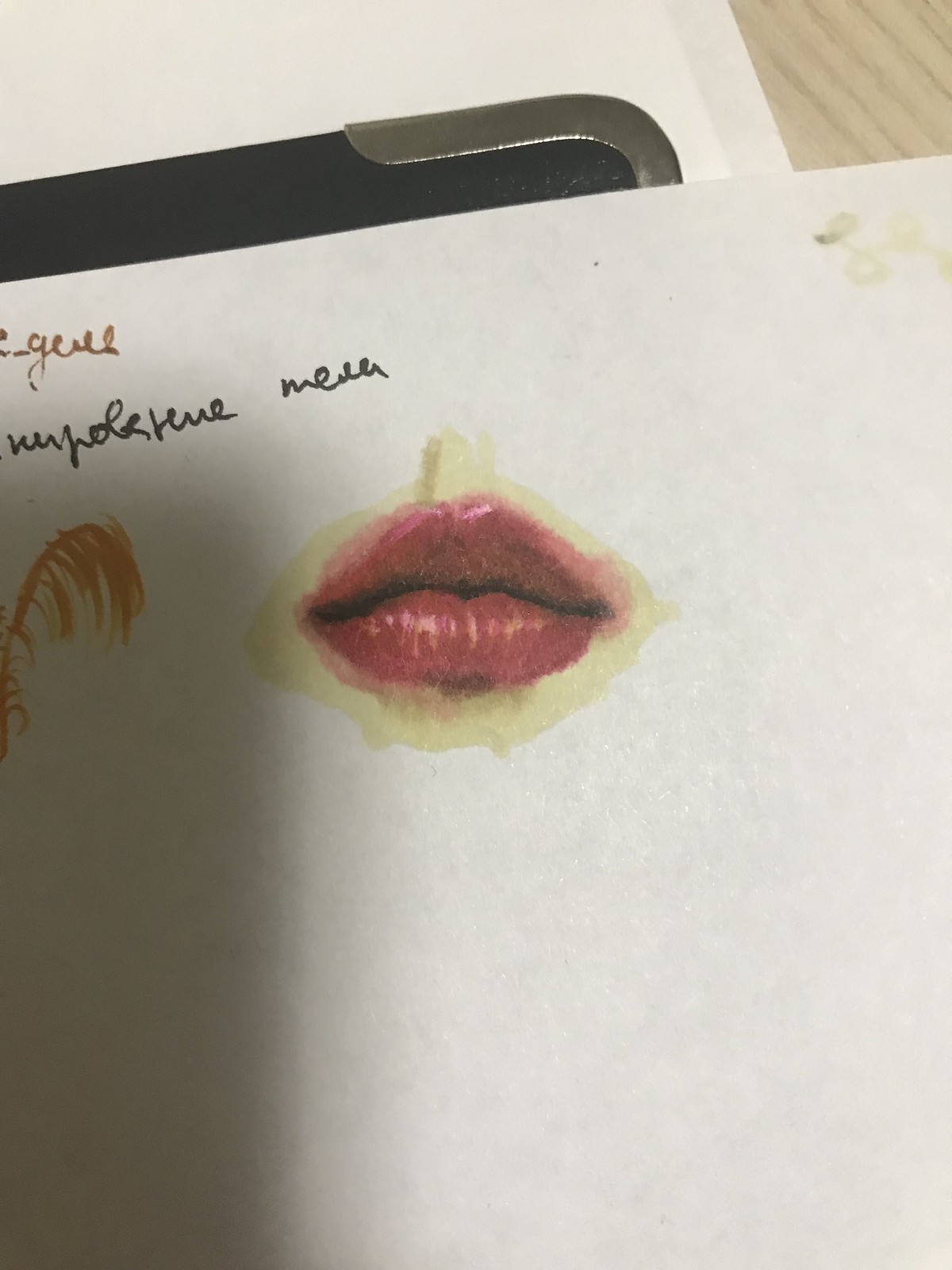The image depicts a detailed painting of vibrant red and black feminine lips on a white piece of paper. Surrounding the lips is a subtle, yellowish or vanilla-tinted border. To the left of the lips, there is a small, doodle-like sketch featuring orange lines or perhaps a feather. Above the painted lips are two lines of text: the lower line in black ink and the upper line in a darker orange or brownish ink, which seems to be in a non-English script. This centerpiece paper is placed on top of a black notebook or similar object, identifiable by its silver lining at the upper right corner, and the entire composition is set against another white surface that rests on a wooden panel.